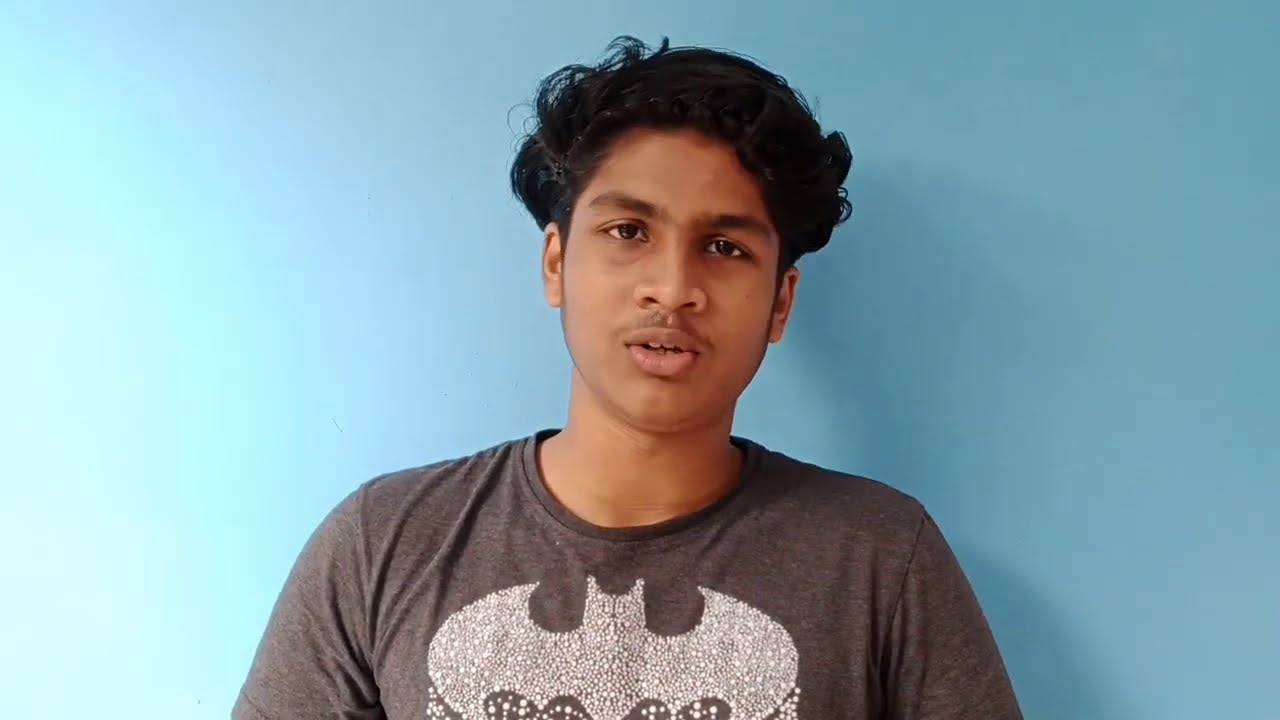The image features a young male, likely in his mid to late teens, with light brown skin, possibly of South Asian or Indian descent. He is captured standing against a wall that transitions from a very light blue on the left to a darker light blue on the right. The lighting source from the left casts a slight shadow over his right shoulder. He has wavy or curly black hair that is longer on the top and off his ears, as well as a developing mustache and a faint unibrow. His head is slightly tilted toward the right, and he appears to be talking to the viewer, suggesting this might be a still frame from a documentary or an interview. He is wearing a heather gray short-sleeved t-shirt that fits a bit loosely. The shirt prominently features the Batman symbol, which is composed of small white dots, giving a distinct beaded appearance.